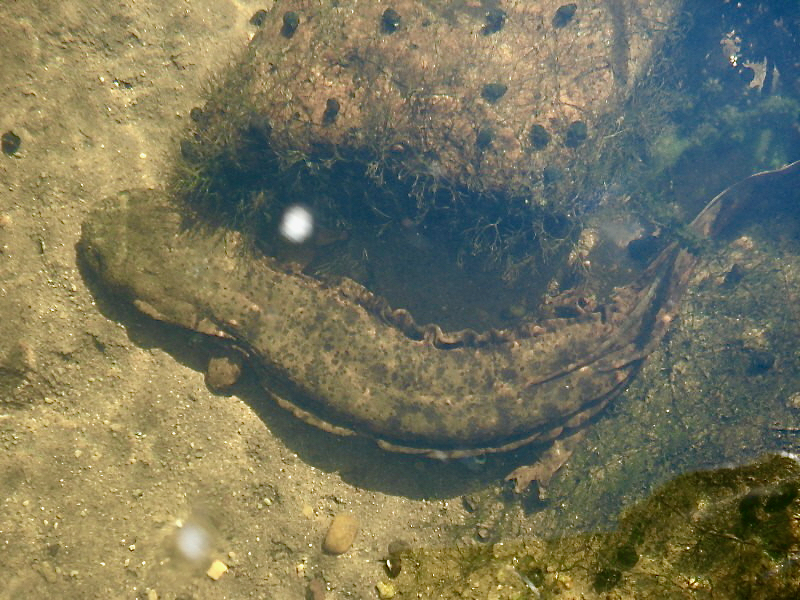This underwater photograph captures the serene scene at the bottom of a riverbed. Dominating the center of the image is a catfish, approximately a foot long, resting on the sandy and rocky river floor. The catfish is covered in moss, with small pebble-like growths adorning its back, and appears to be one of those species that uses a bright lure to attract prey. Surrounding the catfish are various sizes of rocks, ranging from small pebbles to larger stones, accentuating the complex textures of the riverbed. Interspersed among the rocks are patches of green, likely aquatic plants or grasses, adding a touch of color to the predominantly brown and earthy tones of the scene. Near the bottom of the frame, there appears to be a long, eel-like creature with a broad head, similar to an alligator or lizard, showcasing short, stubby limbs and tapering into a slender tail. This well-composed image highlights the rich and diverse micro-ecosystem thriving at the river's bottom.